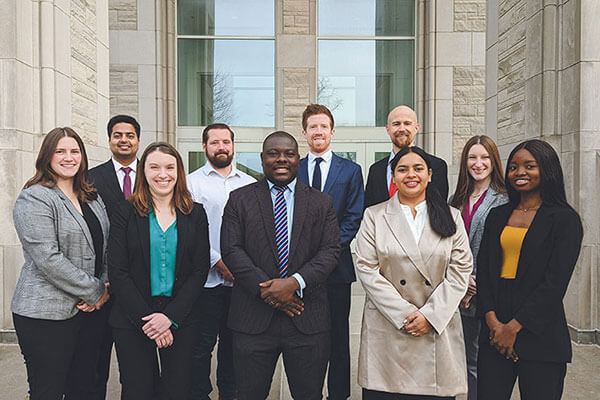The image depicts a group of ten professionally dressed individuals standing in front of a building with a white, possibly beige stone exterior and large windows that show reflections of leafless tree branches. The group is arranged in two rows, with the shorter row in the front and the taller row in the back. The front row consists of six people, predominantly women along with a black man in the center, who is wearing a dark gray suit, a blue and orange striped tie, and a light blue shirt, and has his hands crossed while smiling. The woman second from the right in the front row is notably dressed in a raincoat. The back row features four men, mostly in suits; one man, second from the right, is not smiling. All individuals appear to be between their late 20s and early 40s. Most of them are smiling and exhibit a blend of business and business casual attire with blazers and ties being prominent among the men, indicating a professional setting potentially outside a government building, law office, or courthouse.